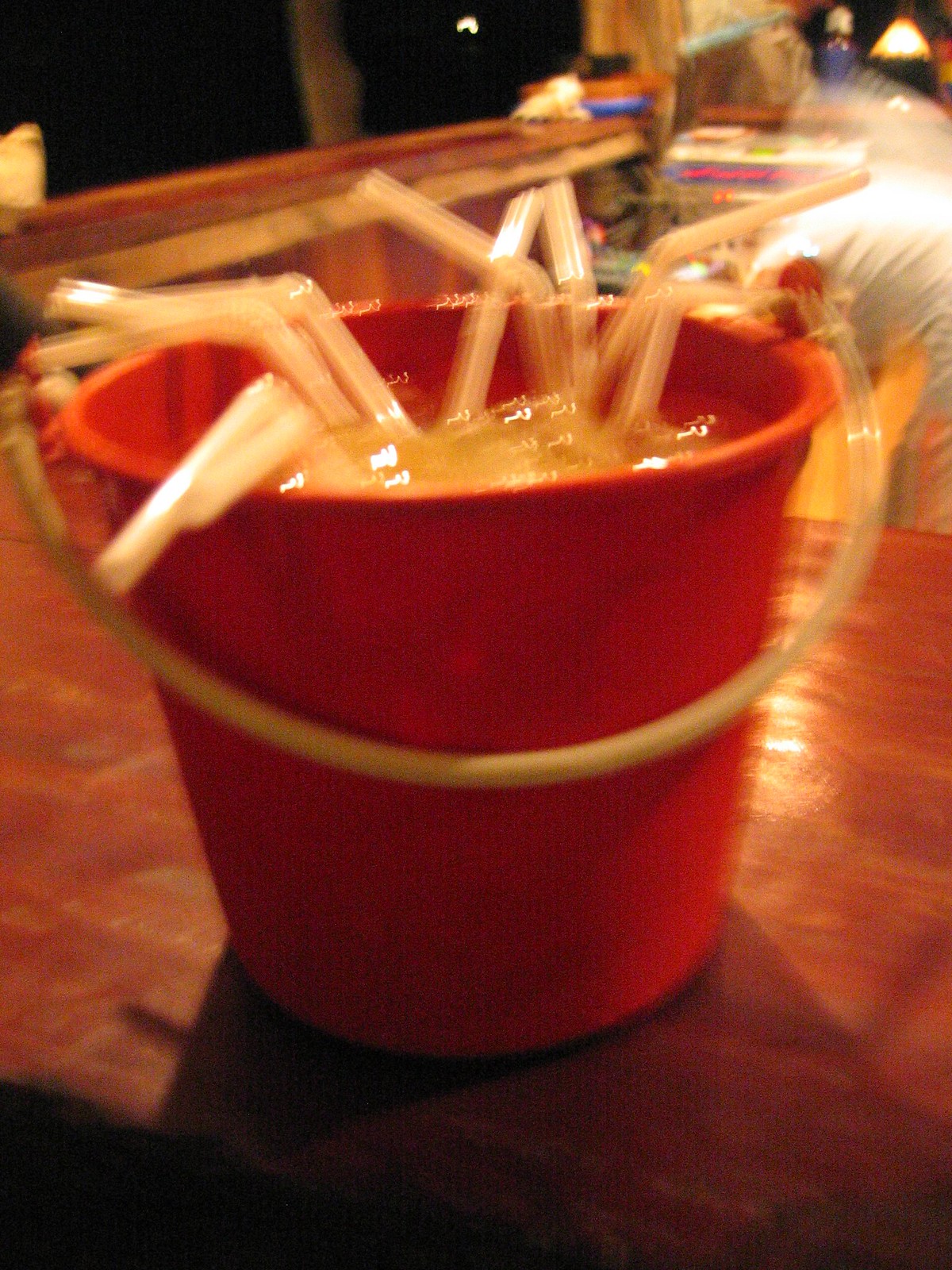The image is a color photo that is extremely out of focus, making it difficult to discern all details clearly. At the center, there is a red plastic bucket with a white handle folded down, reminiscent of the buckets used by children for building sandcastles. The bucket appears to be filled with a yellowish drink, complete with ice, and has eight to ten drinking straws sticking out of it, some of them having an accordion-like bend. The straws are overlapping and draping over the side of the bucket, giving it the look of a communal drink designed for sharing among several people.

The bucket is placed on what seems to be a brown wooden table. To the right side of the bucket, there's a faint and indistinct presence of a hand wearing a white glove. The background reveals components of an outdoor setting at night, highlighted by bright lights shining down, creating glares. At the top left corner, a narrow countertop covered in the same surface as the table can be seen. Additionally, features like a large double window and what might be a bench, along with indistinct hues of white and purple, add context to the otherwise blurry and unfocused image. The brick-like surface beneath the bucket and the blurred elements contribute to the overall uncertainty about the exact setting, though it appears to be an outdoor or partially outdoor space.